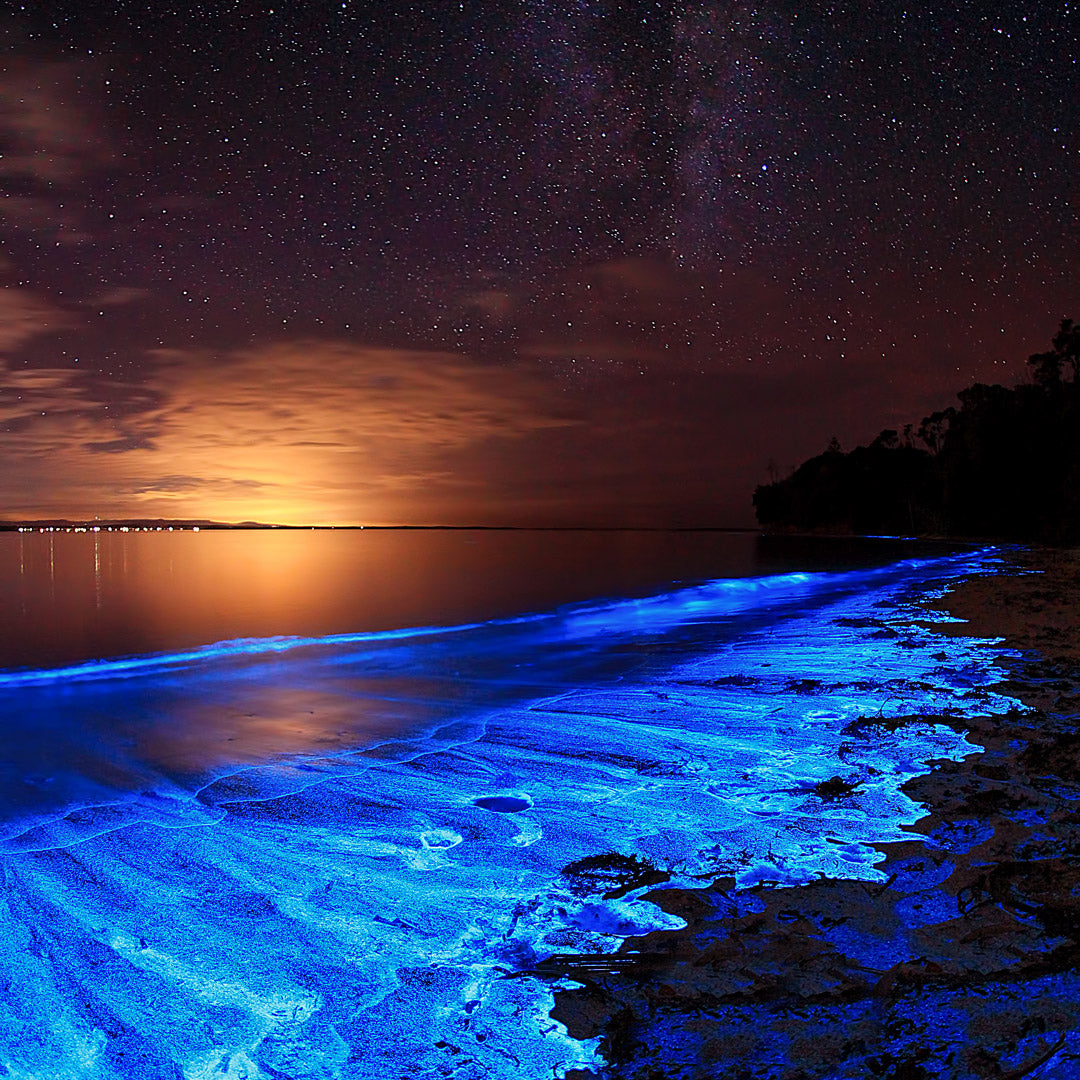This image captures an artistic rendition of a serene seascape at nighttime, possibly during evening dusk given the setting sun in the background with its orange reflection across the calm, dark waters. The sky is a mesmerizing tapestry densely packed with stars, creating the impression of an untouched, remote area. A faint purple hue adds depth to the celestial panorama. This beach scene is characterized by bioluminescent waves, their bluish glow delineating the shoreline and adding an ethereal quality to the small cove. The foamy waves gently lap against the right side of the beach, where trees and a bit of sandy shore are discernible. In the distance, lights from buildings on the other side of the water suggest a distant city on the horizon. The colors in this scene blend beautifully, with shades of blue, orange, black, and white harmonizing to create a captivating and tranquil nightscape.